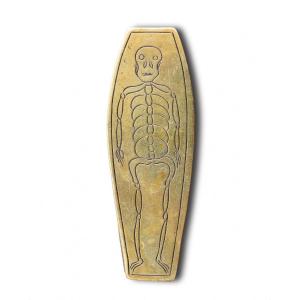The image showcases a small, flat, coffin-shaped artifact with a bony, yellowish golden bronze color, displaying an older, tarnished quality. Engraved on the object is a simple, almost cartoony skeleton, featuring a skull, shoulder and arm bones, spine, ribs, pelvis, leg bones, and feet. The skull appears a bit oddly shaped, potentially representing a non-human primate or animal. The piece is edged by a basic etched border and lies on a plain white background with a slight shadow on the right side. There are no other objects in the photograph to provide a sense of scale, and no text is present.